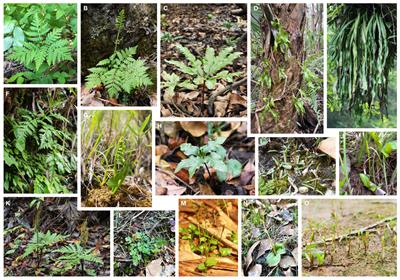The image is a detailed collage consisting of 15 small rectangular photographs, each framed with a white border and labeled with letters starting from A. The entire collage is rectangular in shape and showcases various types of foliage, focusing on different kinds of plants in muted yet clear tones. Among the depicted plants, several on the left-hand side are bright green ferns, while others feature marsh grass and trees with vines entwined around them. The colors range across green, brown, orange, gray, black, and white, with shades of green and yellow diversely represented. Each photograph positions the plant centrally, providing a clear view that resembles a layout one might find in a nature handbook or botanical guide. The photographs collectively offer a vivid display of plant diversity, with each example varying in type and size, from tall branching plants to those with long leaves extending towards the ground.